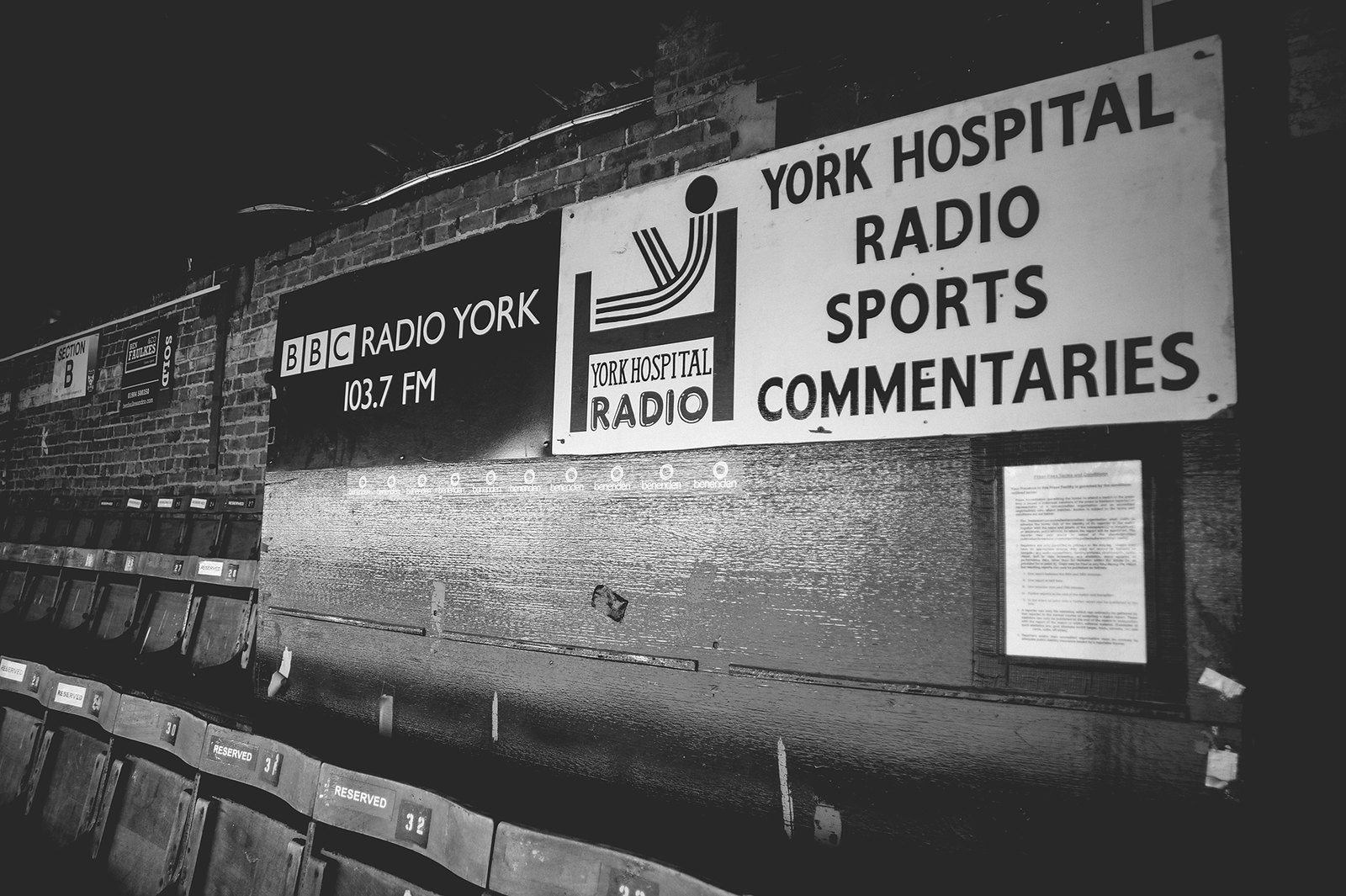The black and white photograph depicts the interior of a sports stadium. At the bottom left, rows of numbered seats extend diagonally, each marked with the word "Reserved." The seats, such as those numbered 30, 31, and 32, appear folded up. The highest row of seats is set against a brick wall that forms the backdrop of the image. On the far left side of the brick wall, there is a sticker or a poster indicating "Section 8." Dominating the middle portion of the image, two advertisements are affixed to the brick wall. The left advertisement, set on a black background with white text, promotes BBC Radio York 103.7 FM. The advertisement on the right, featuring black text on a white background, is for York Hospital Radio Sports Commentaries, with the York Hospital Radio logo on the left. Beneath these banners, a framed piece of paper with smaller, illegible printing can be seen. Overall, the image captures a section of the stadium characterized by its brick construction and promotional materials for local radio stations.